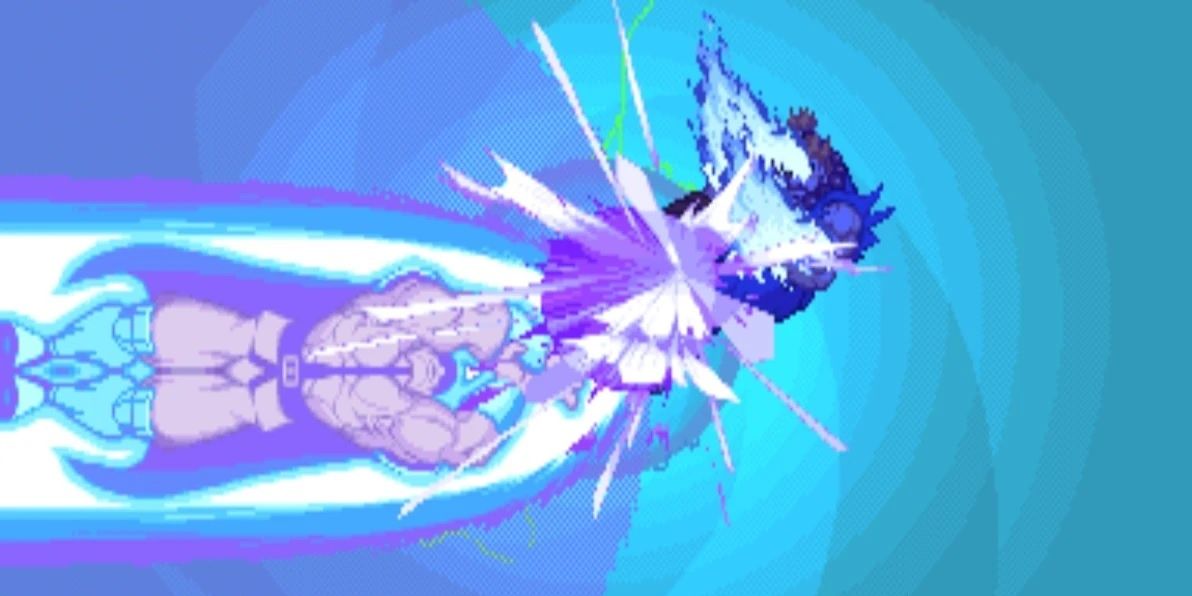The image depicts a dynamic and abstract scene, likely from a video game or graphic illustration. Dominated by shades of teal blue and a bluish purple, the background is textured and features bright white light emissions. To the left side of the image stands a large, muscular superhero character with a long, thin beard and black hair. He's notably shirtless, wearing bright blue pants, blue boots, blue cufflinks around his wrists, and a black belt. The superhero appears to be generating a powerful energy wave or handling a significant explosion of bluish-purple hues above his head. The scene is rotated horizontally, adding to the abstract feel, and suggests the superhero might be smashing through ice or water, creating cracks and scattering shades of blue and purple. The image conveys a sense of strength and action, emphasizing the superhero's powerful presence amidst a burst of energy.